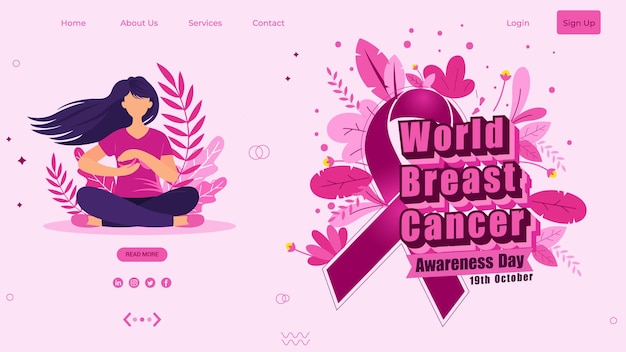On World Breast Cancer Awareness Day, the image features a predominantly pink theme to symbolize support and awareness for breast cancer. The background is pink, matching the pink text and a darker pink awareness ribbon prominently displayed. At the top of the image, navigation options include "Home", "About Us", "Services", "Contact", "Login", and "Sign Up". 

The focal point of the image is a woman seated with her legs crisscrossed, gently cupping her right breast with her hands, symbolizing self-examination and awareness. She has long black hair and is dressed in a pink shirt, black pants, and pink shoes. Surrounding her are pink-leaved plant ferns, adding to the supportive and caring atmosphere of the image.

Below her, the text "Read More" invites viewers to further engage with the content. Social media icons for Twitter, Facebook, Instagram, and a yet-to-be-identified square platform are displayed beneath this call to action. Further down, two arrows with three pink dots in between them hint at additional navigational options or content.